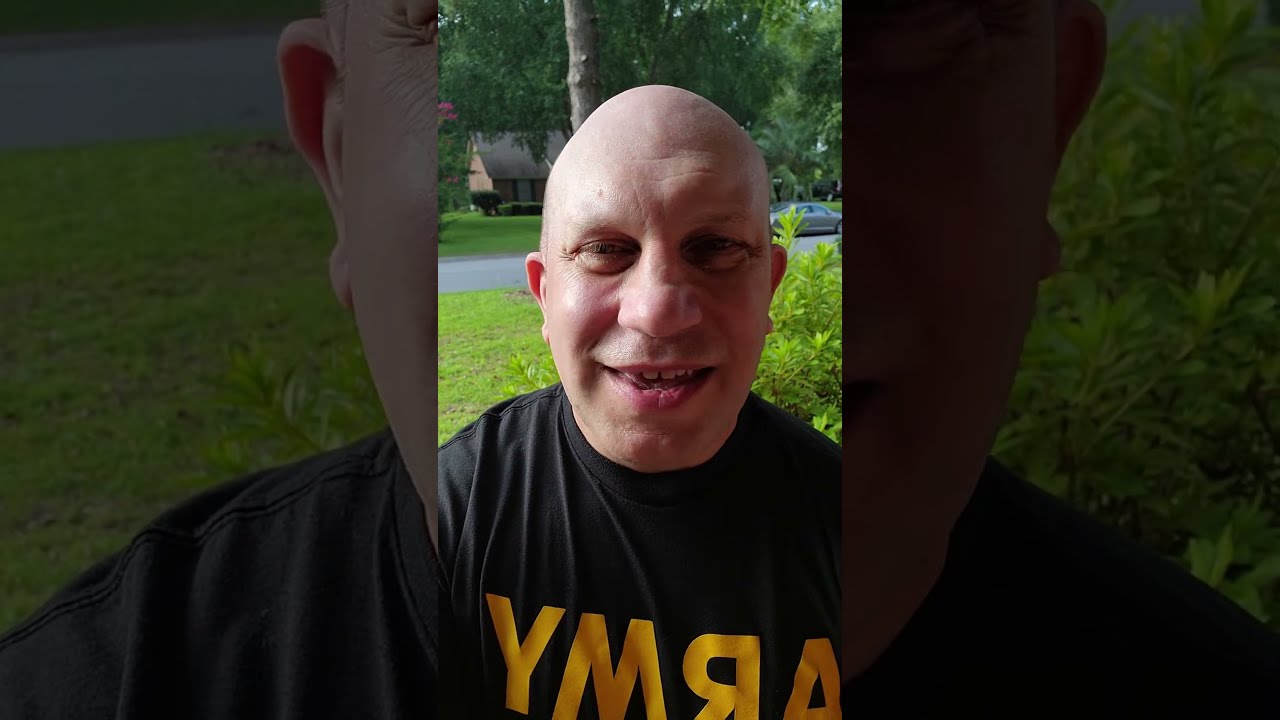The image is a wide rectangular photograph set against a solid black background on both sides. At the center stands a vertically oriented, detailed picture of a middle-aged, bald man with light skin and distinctive facial features, including barely visible eyebrows and spaced-apart teeth. He appears to be smiling widely with his mouth open. The man is wearing a black t-shirt with the word "ARMY" emblazoned in large, yellow block letters, though the text appears reversed in the image. The background depicts a suburban outdoor setting with a bright green lawn and bushes on either side of him, a gray road at the top of the image that slopes slightly upward, and a silver car parked on the right side of the road. Beyond the road, there's a darker green lawn, a tall brown house with a triangular roof, and a tall tree, contributing to the snapshot of residential tranquility.